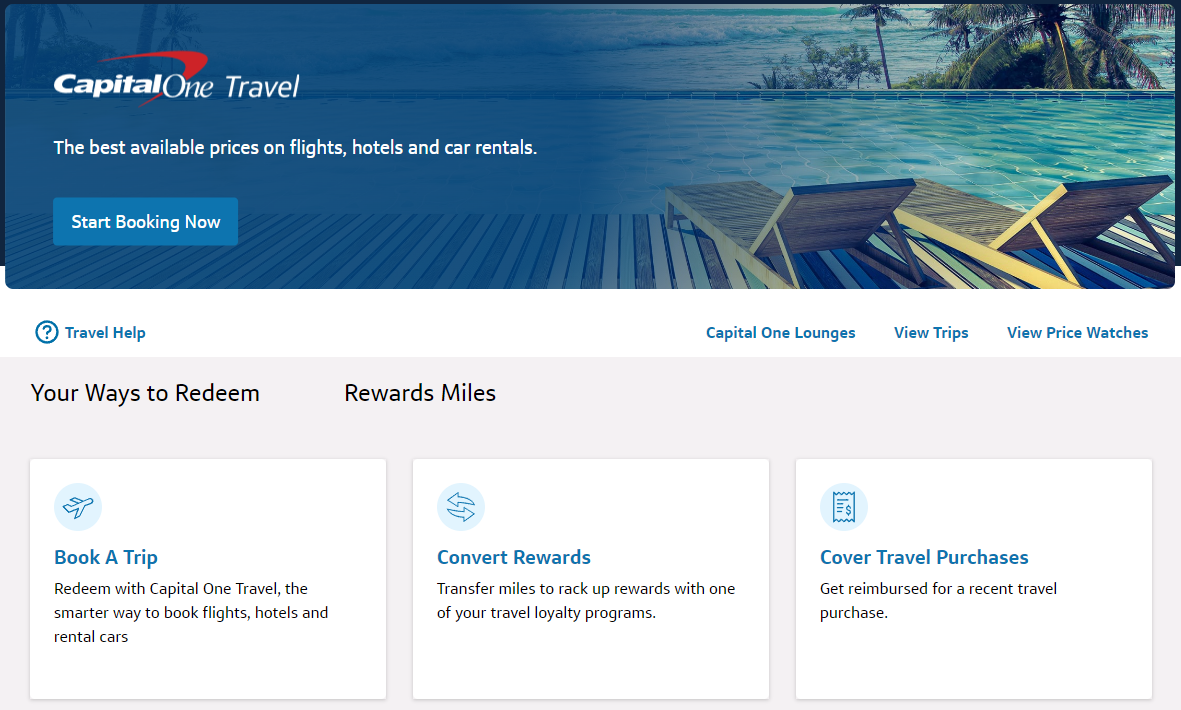The homepage image of Capital One's travel website reflects a serene tropical ambiance, featuring a pool and two deck chairs overlooking a beach reminiscent of Hawaii. The top-left corner displays the iconic Capital One logo, characterized by its familiar red arc behind the "Capital One" text. Adjacent to this logo, the word "Travel" is prominently displayed in a crisp white font. Below the logo and added text lies the company’s slogan: "The best available prices on flights, hotels, and car rentals."

A prominent call-to-action button, set within a contrasting blue box with white text, encourages users to "Start Booking Now." The top menu, seamlessly overlaid on the idyllic background image, offers various navigation options for the users. Scrolling further down the page presents an array of user-friendly features and hyperlinks, such as "Travel Help" for personalized assistance, "Capital One Lounges" for exclusive travel experiences, "View Trips," "View Price Watches," and tabs indicating ways to redeem rewards, including "Reward Miles" and "Reward Points." These elements aim to provide an intuitive and comprehensive travel booking experience integrated deeply within the Capital One ecosystem.